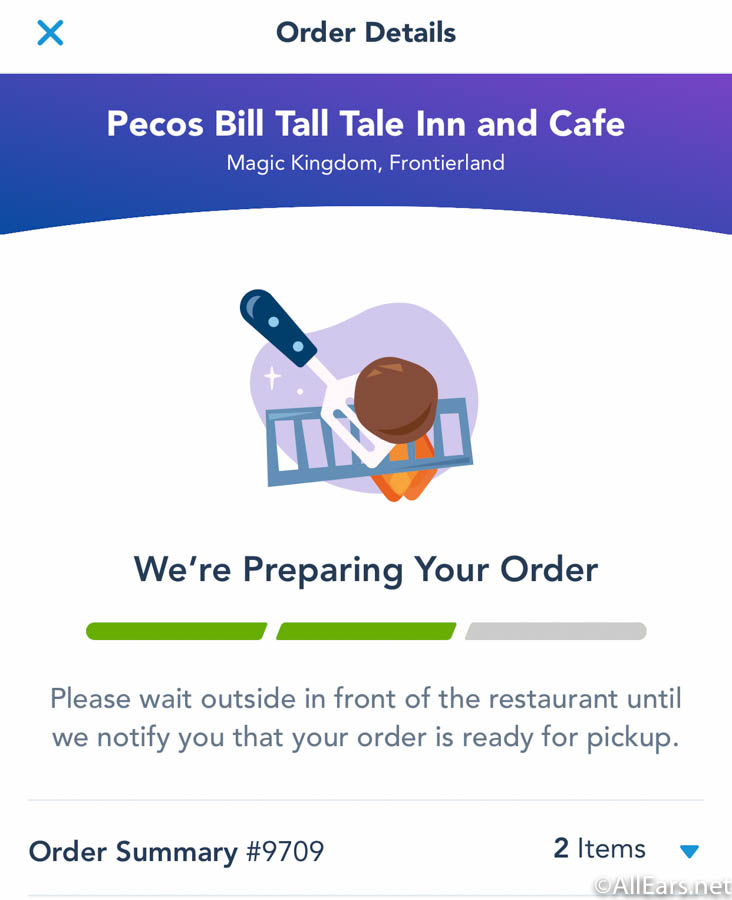The image features an order summary from a restaurant. Positioned in the top left corner, text in blue reads "Blue Axe." Directly below, larger blue text displays "Order Details." The document is set against a white background. 

In the top-right section, the text indicates the establishment's name: "Pecos Bill Tall Tale Inn and Cafe," located in "Magic Kingdom, Frontierland." Below this header, there are illustrations of a grill, a spatula, a meat patty, and flames indicating food preparation.

The text instructs patrons to "Please wait outside in front of the restaurant to notify the order as we pick up your order." It provides an "Order Summary number 9709" and lists "two items."

Additional details include a copyright notice attributed to "All Your Restaurant" and various decorative lines, enhancing the structured appearance of the order summary.

In terms of color, the main text is green with some elements in grey. Noteworthy visual elements include a purple and blonde motif, possibly part of the restaurant's branding or theme.